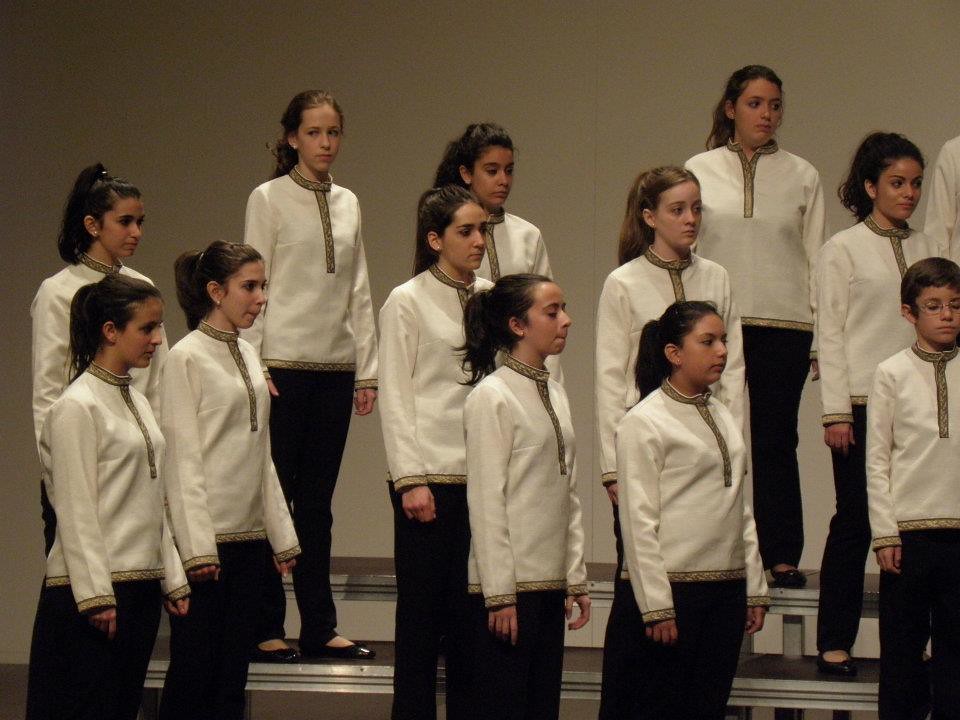The image portrays a chorus of mostly teenage girls, with one boy standing on the far right. They range in age from approximately 12 to 16 years old. Everyone is dressed uniformly in black pants and white long-sleeve shirts, adorned with brown or gold trim that runs from the collar down to the mid-chest. Despite their uniform look, one girl stands out by looking directly away from the group, whereas most others are facing to the right, with some glancing around. The boy on the right dons glasses and has short hair, with his eyes closed. The group is positioned on metal bleacher-like steps, set against a brownish-gray wall background, lending an organized and structured appearance to their formation. The girls predominantly have their hair in brown ponytails and are all wearing black shoes.